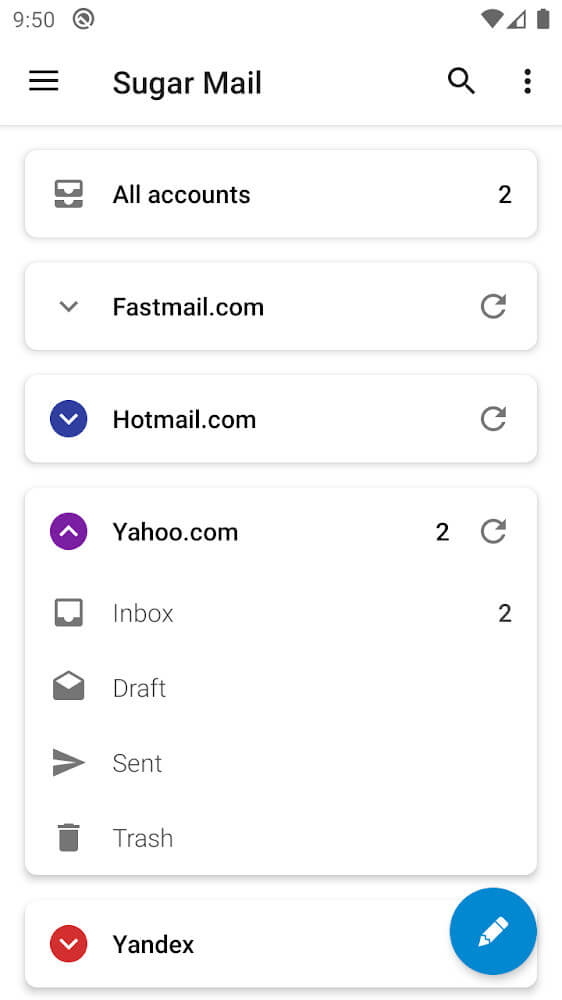The image is a screenshot of a mail application displayed on a smartphone in portrait orientation. The top-left corner shows the time as 9:50, while the top-right corner indicates that the battery is nearly full. The app is identified as "Sugar Mail" at the top of the screen, accompanied by a hamburger menu icon on the left for additional options, a magnifying glass icon in the middle for searching, and a vertically-stacked three-dot icon on the right for more settings.

Below the app's title, "All Accounts" is listed with an icon indicating two accounts in total. The first account is labeled "fastmail.com," featuring a refresh button to the right. Following it is "hotmail.com," and then "yahoo.com," where the number '2' on the far right indicates the presence of two unread messages or new items associated with this account.

A categorized breakdown of the "yahoo.com" inbox shows two items in the inbox, with no items in drafts, sent, or trash folders. The bottom section of the screen briefly mentions another account, "Yandex," although there is no additional detail provided about it.

In the bottom-right corner of the screen, there is a prominent blue circle icon featuring a pen, likely representing a button to compose a new email.